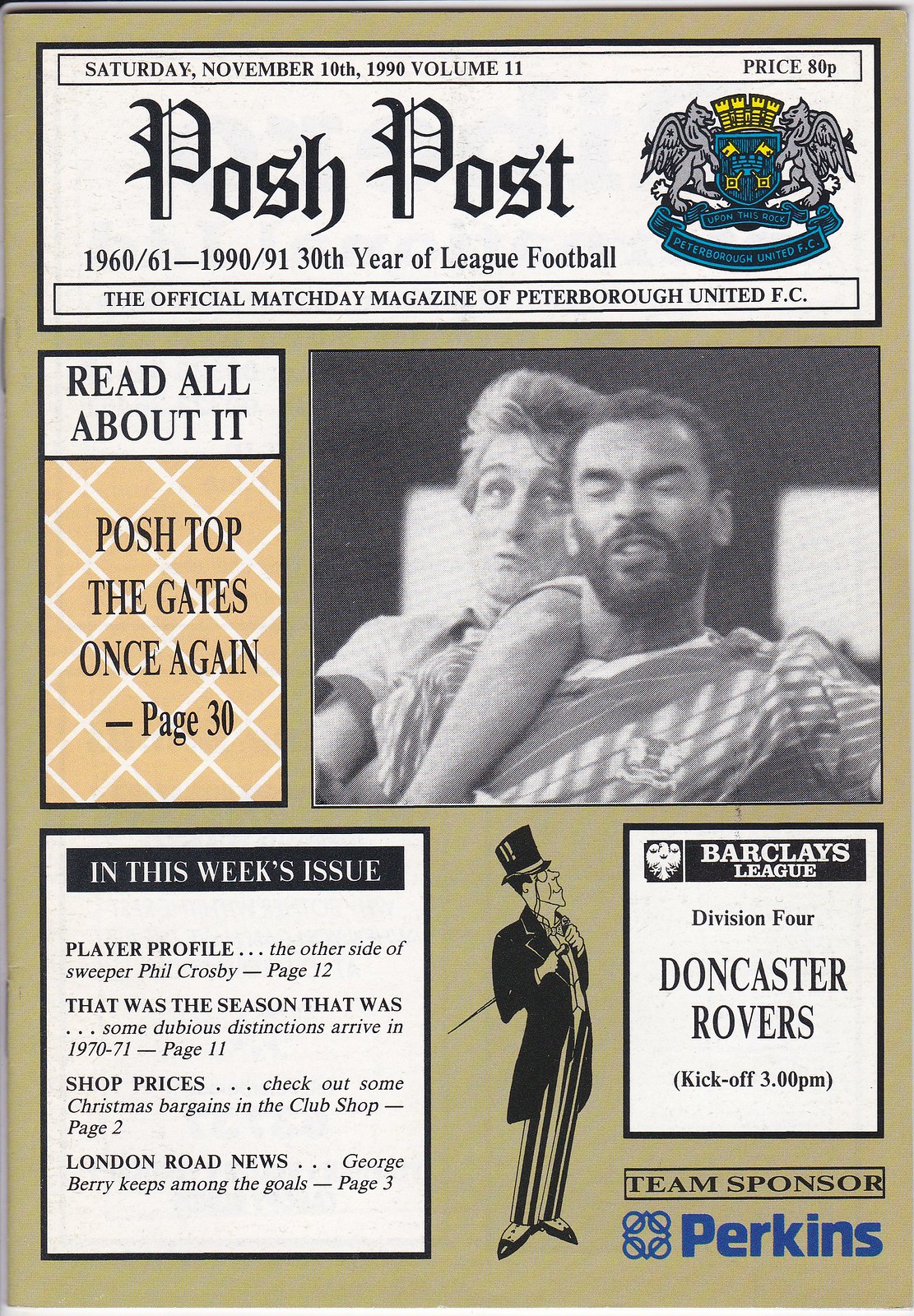The image is of a digitally designed magazine cover, specifically the official match day magazine of Peterborough United FC. The cover has a beige or tan background, and at the top, there is a banner with the title "Posh Post" written in italic script, indicating it commemorates "1960 to 61 to 1990 to 91: 30th Year of League Football." In the upper right corner, a crest featuring a shield flanked by two winged lions is displayed. 

Below the banner, there is a small vertical rectangle with text reading "Read all about it. Posh tops the gate once again page 30." To the right of this box is a black and white photograph of two soccer players, both seen from the torso up, one with his arm around the other, and both making faces, with one player's eyes closed. 

In the lower left corner, a smaller vertical square contains the words "In this week's issue" followed by additional text. The center bottom of the cover features a caricature of a man in a top hat and tails. In the lower right corner, a small square announces "Barclays League Division 4: Doncaster Rovers kickoff 3 p.m. Team sponsor Perkins." Additional text mentions "Saturday, November 10th, 1990, Volume 1, Price 80p."

The overall color scheme includes beige, black, white, teal, and yellow.